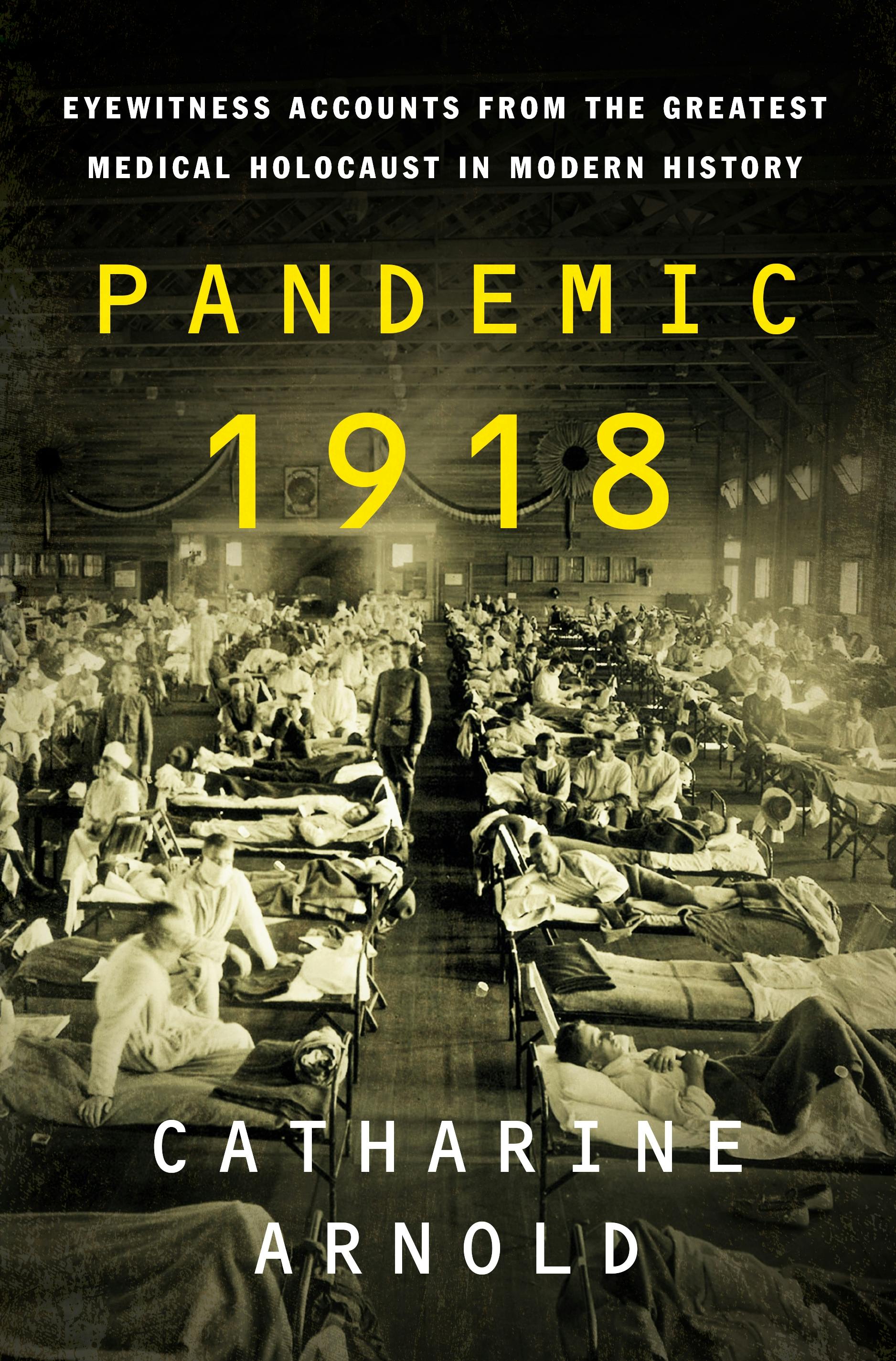This image is the front cover of a book, presented in portrait orientation and measuring approximately six inches high by three inches wide. The top of the cover features a caption in small white letters: "Eyewitness Accounts from the Greatest Medical Holocaust in Modern History." Beneath this, the book's title "Pandemic 1918" is prominently displayed in larger yellow or gold letters. At the bottom, "Catherine Arnold" is written in white.

The background of the cover transitions from black at the top to a vintage black and white photograph occupying the majority of the space. This photograph depicts the interior of a large clinic or hospital ward during the 1918 influenza pandemic. Multiple rows of twin-sized beds or cots are shown, densely packed with patients, some lying down and others sitting up. A light tan glow highlights the center of the image, drawing attention to the sheer number of bedridden individuals. Notably, some patients and doctors are wearing masks, although not everyone adheres to this precaution. Most patients appear to be male, and linens are scattered around the cots. The overall scene conveys the gravity and scale of the medical crisis depicted within the book.